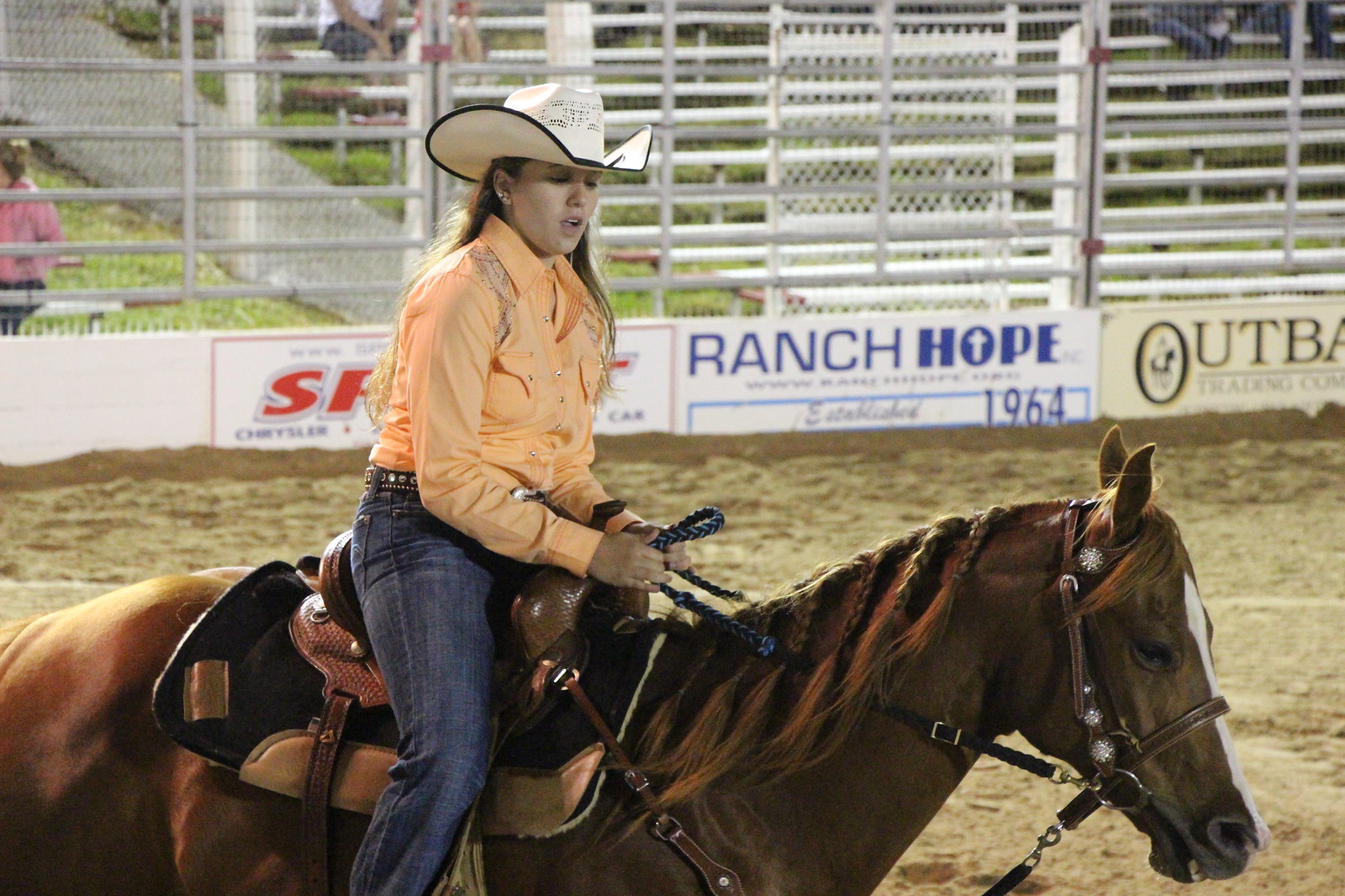The image depicts a woman riding a brown horse with a distinctive white stripe running from the middle of its eyes to the tip of its nose. The horse's mane is braided, almost resembling pigtails, and it has blue reins in its mouth with its top teeth slightly protruding. The woman, slightly heavier than average but not quite fat (an American XL size), has long dirty blonde hair and is adorned in a white cowboy hat with a black rim. She's dressed in a light orange, slightly see-through, long-sleeved collared button-up shirt and is wearing blue jeans with a black studded belt. The saddle she sits on is predominantly black, featuring brown leather on the top and light beige leather on the bottom edges. 

They are situated in a patch of sand, surrounded by a tall white fence made of steel with a solid base where numerous sponsor advertisements are visible. Notable signs include "Ranch Hope 1964" and another with partial red writing showing the letters "S" and "P." Despite the intricacies of the scene, it's a bright and pleasant day, adding to the overall picturesque quality of the photograph.